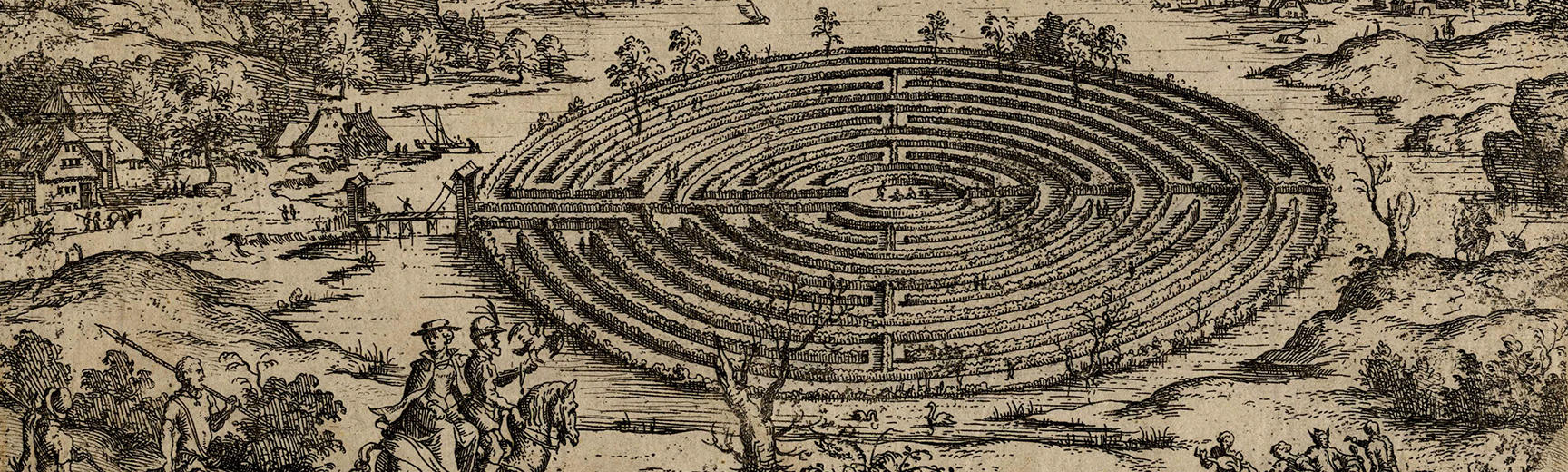This image is a detailed, rectangular ink drawing set on a light, tannish beige background, depicting a scene from an older period, likely the 19th century. The central feature is a large circular maze with concentric paths suggestive of it being constructed from rocks or plants. In the very center of the maze, a couple of people are visible, and more figures are scattered throughout the pathways.

On the left side, an entrance to the maze can be seen, accessible via a small bridge crossing a body of water. Adjacent to the bridge, there's a small town area with old English-style buildings and a backdrop of rolling hills and sparse trees.

At the forefront in the lower left corner, the scene becomes more animated with several people depicted: two individuals are riding a horse, a man is holding a long spear on his left shoulder, and a few others are walking. The edges of the image are adorned with additional trees, branches, and bushes, contributing to a sparse yet intricate landscape. The overall artwork exudes a sense of historical outdoor activity within a structured labyrinthine environment.